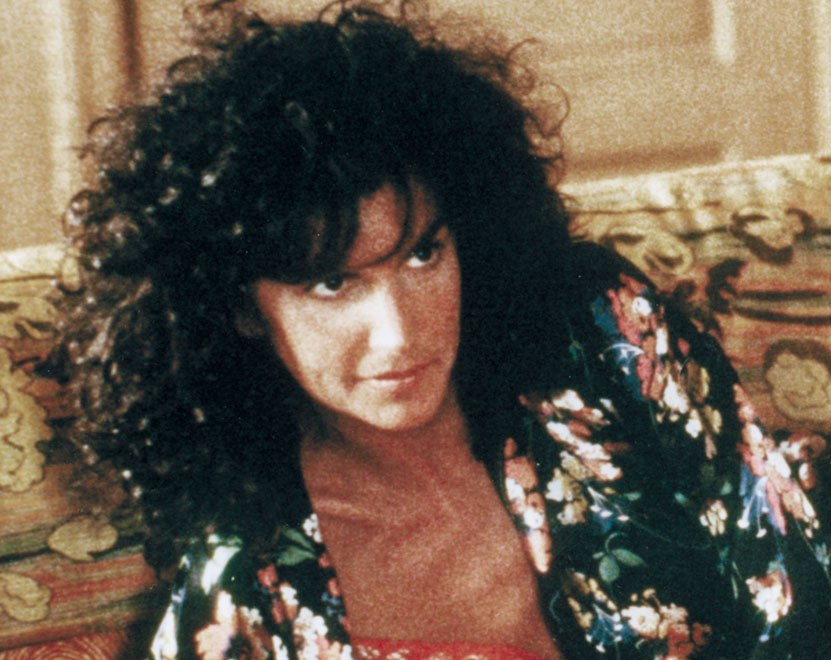The photograph, reminiscent of a movie still, features an attractive actress from the 80s or early 90s who looks vaguely familiar. She has thick, long, and unruly black hair with bangs over her forehead. Dressed in a floral print silk bathrobe that's open to reveal a red silk negligee underneath, she exudes a seductive aura. The actress, with dark eyebrows and intently listening or looking towards somebody off-camera to her right, is seated on a floral-patterned sofa. The sofa itself boasts a mix of greens, reds, pinks, and a tan color. The background showcases a beige door and wall, complemented by white curtains and tight beige pipes. This detailed scene captures a moment of intense focus and allure.